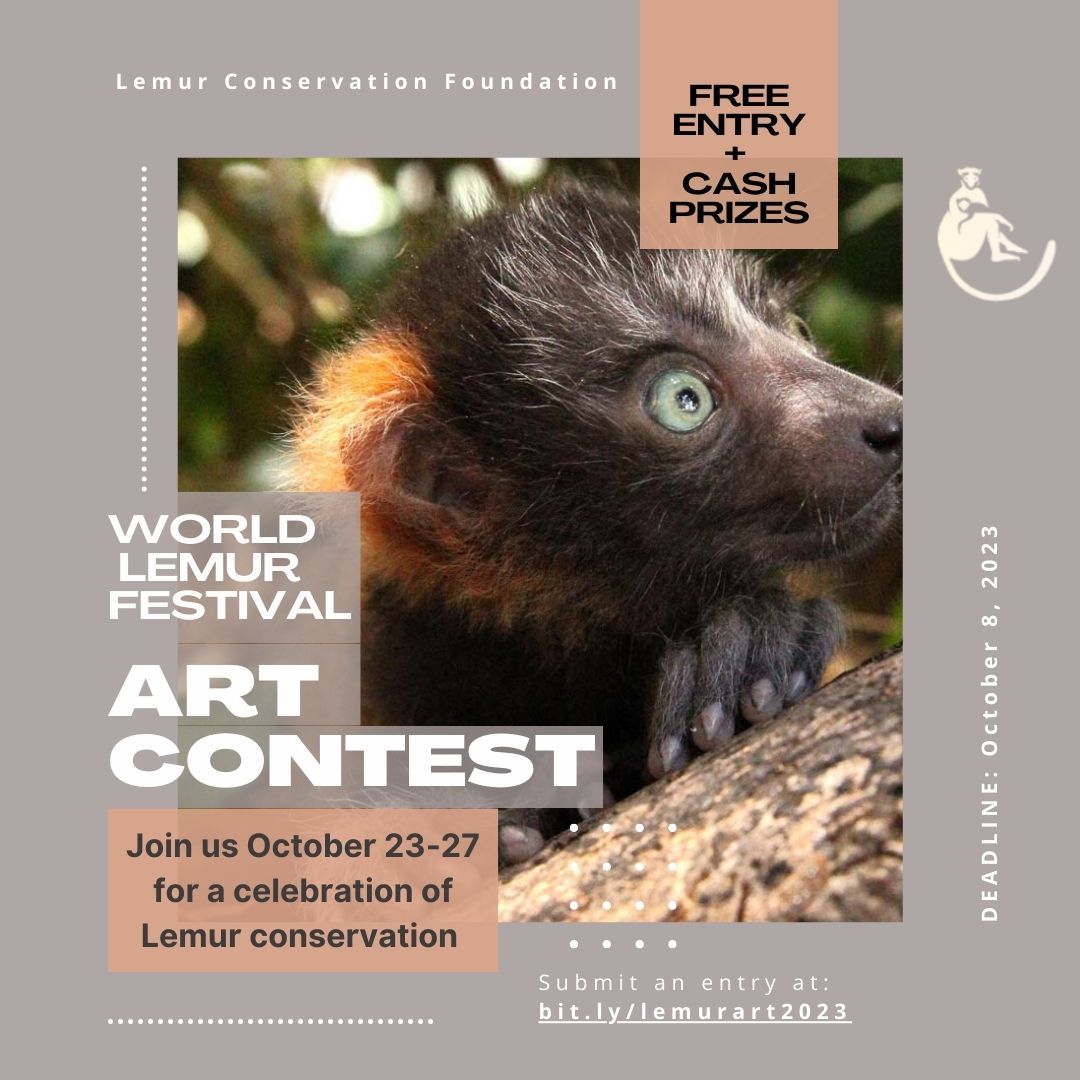The poster for the "World Lemur Festival Art Contest" prominently features a closely cropped image of a lemur with green eyes and brown fur, resting one paw on a tree trunk. The background is filled with out-of-focus foliage, adding depth to the image. The poster has a light gray border with white and black text, and an orange-pink highlight box at the top. Key information outlined includes the event dates, October 23-27, and the submission deadline of October 8, 2023. The text also mentions "Lemur Conservation Foundation" at the top, and highlights the benefits of free entry and cash prizes. An illustration of a mother lemur holding its child is also incorporated in the design. Additional submission details and instructions are provided at the bottom, including a link: bit.ly/lemurart2023.